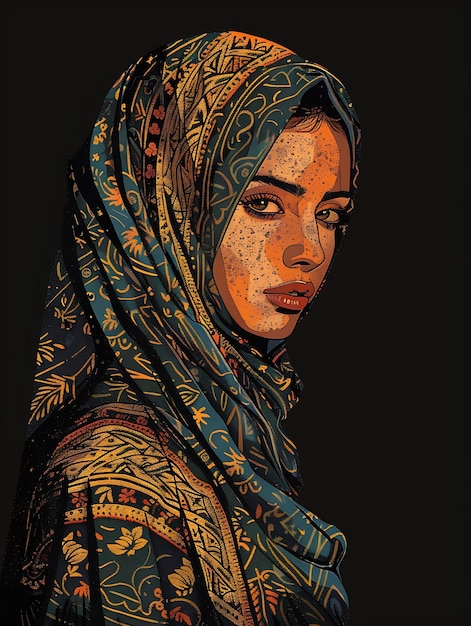This image, likely a painting or a highly stylized digital illustration, depicts a woman gazing directly at the viewer with a soft, penetrating look. Although her body is partially turned to the right, her eyes remain fixed on the viewer, creating an engaging and intimate portrait. She is adorned in a beautifully detailed headscarf, also known as a hijab, featuring an intricate pattern with shades of deep blue-green, blue-gray, gold, and tan. The design is adorned with motifs resembling wheat, flowers, pine needles, leaves, stems, and crisscross geometric patterns. Her blouse mirrors this exquisite print, suggesting a cohesive traditional ensemble, possibly akin to a sari. The woman's dark hair peeks out subtly, and her lips are enhanced with lipstick, adding to her striking appearance. Her complexion shows delicate speckles that resemble freckles, adding to the naturalism of the portrait. Set against a stark black background, the artwork emphasizes her expressive eyes and the vibrant details of her clothing, merging realistic and comic elements to captivating effect.